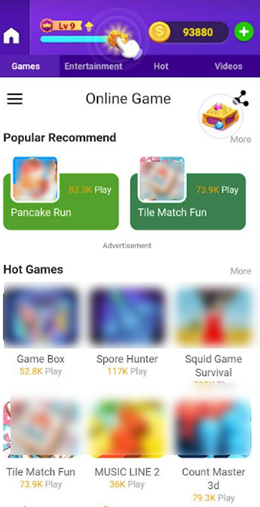The image depicts an open cell phone interface featuring multiple sections and icons. The top portion of the screen is not visible, obscuring any information like the date or time. A prominent purple banner, darker on the left and bottom edges, dominates the view. On the left side of this banner, an icon of a house signifies the home section. Directly beneath, categories such as "Games," "Entertainment," "Hot Videos" are listed; each is associated with an icon, including one showing a white-gloved hand clicked on something above the "Hot Videos" label.

Below this banner, a highlighted tab shows a balance of $93,880, with an adjacent green button for adding funds. Centrally positioned beneath this, a hamburger icon precedes the text "Online Game," accompanied by a share icon. Below this central section, the interface showcases various game listings under two categories: "Popular Recommends" and "Hot Games." "Popular Recommends" features games like Pancake Run and Tile Match Fun. "Hot Games" lists offer titles such as Game Box, Spore Hunter, Squid Game, Tile Match Fun, Music Line 2, and Count Master 3D. The overall layout suggests a keen interest in gaming, with a user-friendly setup encouraging engagement.